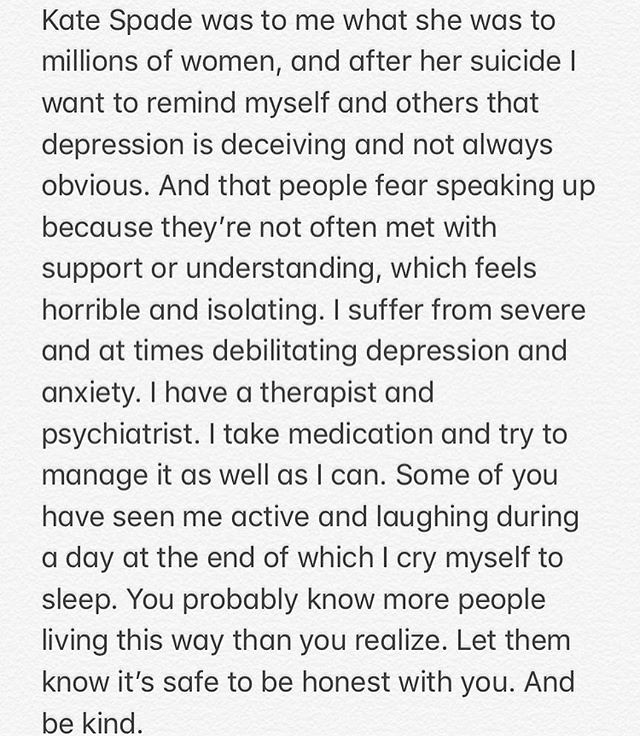This image features a heartfelt, candid message in large black font on a white background, reminiscent of text from Apple Notes. The message speaks to the impact of Kate Spade on millions of women, highlighting the tragic reality of her suicide. It serves as a poignant reminder that depression is often deceiving and not always outwardly apparent, while emphasizing the fear many people have about speaking up due to a lack of support and understanding, which can lead to feelings of isolation. The writer shares their personal struggle with severe and sometimes debilitating depression and anxiety, mentioning that they seek help through a therapist, psychiatrist, and medication. Despite appearing active and cheerful, they admit to crying themselves to sleep, shedding light on the hidden struggles many people endure. The message urges readers to acknowledge the prevalence of such suffering, encouraging them to create a safe, supportive space for honesty and kindness.